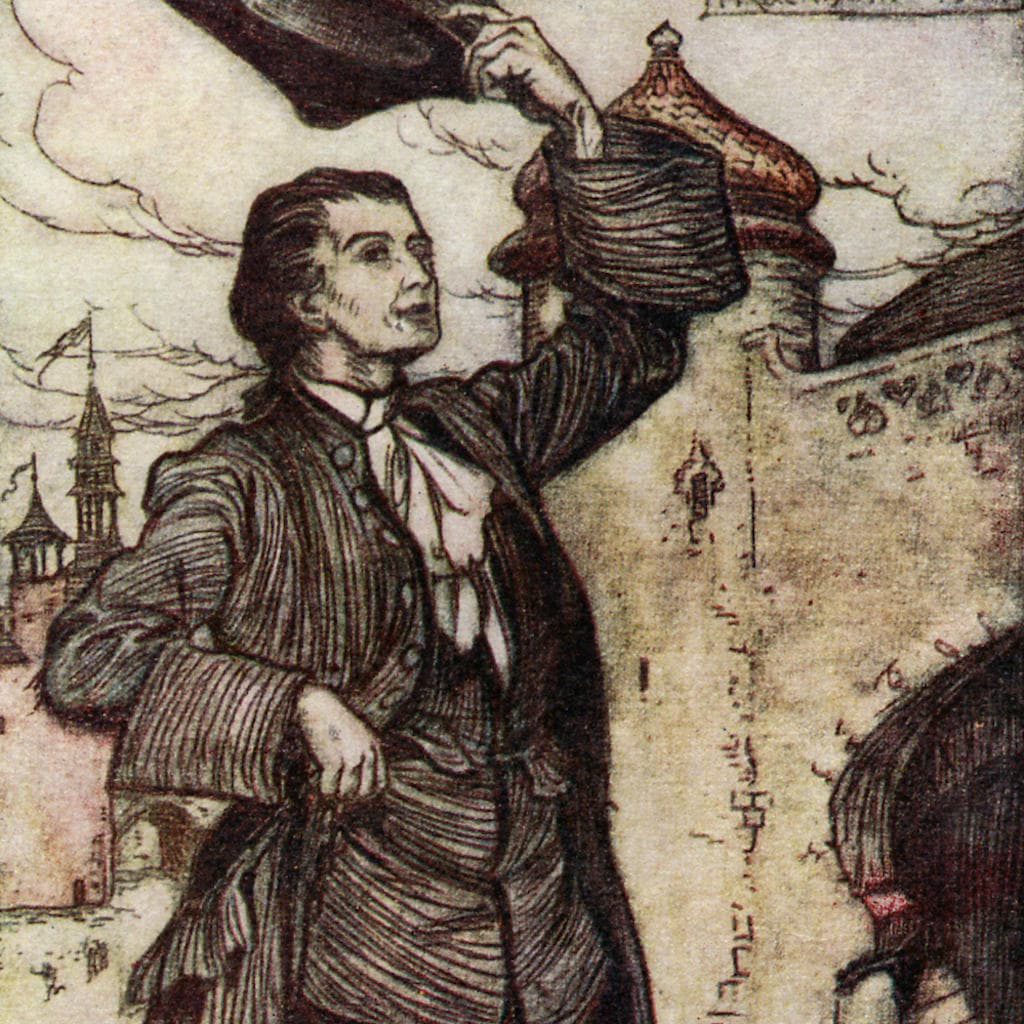This detailed, large square artwork features a brown and light brown sketched drawing, predominantly black and white with touches of color. On the left side, a man from the 1600s stands facing mostly forward while raising a partially visible tri-corner hat in his left hand. He has short, combed-back brown hair and a lightly stubbled face. His attire includes a dark brown jacket with horizontal or vertical lines, featuring exceedingly baggy cuffs. Underneath, he sports a white cravat, extending towards his navel, outlined in brown, and has on a matching vest.

In the background, a light and medium brown stone building with a circular, pointed roof resembling a jar lid dominates the scene. The structure, described as a castle, extends backwards with several visible archways. Above, the sky is filled with dark brown, shaded clouds, drawn in curved lines against a beige backdrop. The upper part of the picture notably includes two narrow towers with flags waving at their peaks. Adding to the lively scene, tiny sketches suggest the presence of people near an archway in the lower left corner, appearing to run towards us.